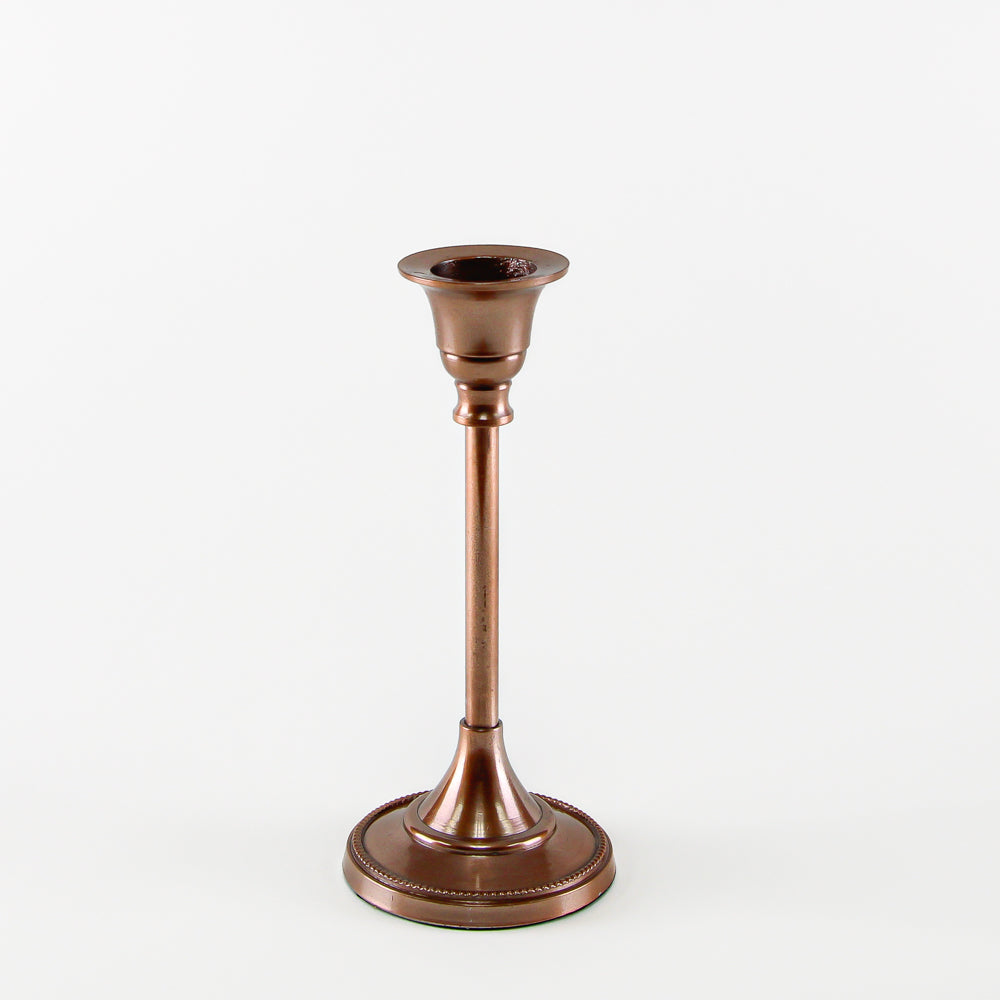This photograph showcases an elegantly designed candlestick holder, crafted from a high-polished metal with a warm, lustrous tone that suggests it may be made of either copper or brass. The holder is specifically designed to accommodate taper candles. Its structure features a wide, round, and thick base that provides stability. From the base, the design ascends into a sleek conical shape, culminating in a slender post. At the apex of this post is an inverted cone, which integrates a cup-like section presumably intended to secure the candle. It is possible that this cup section can be unscrewed from the post, adding a functional element to its intricate design. The combination of refined material and thoughtful engineering makes this candlestick holder both a practical accessory and a piece of art.